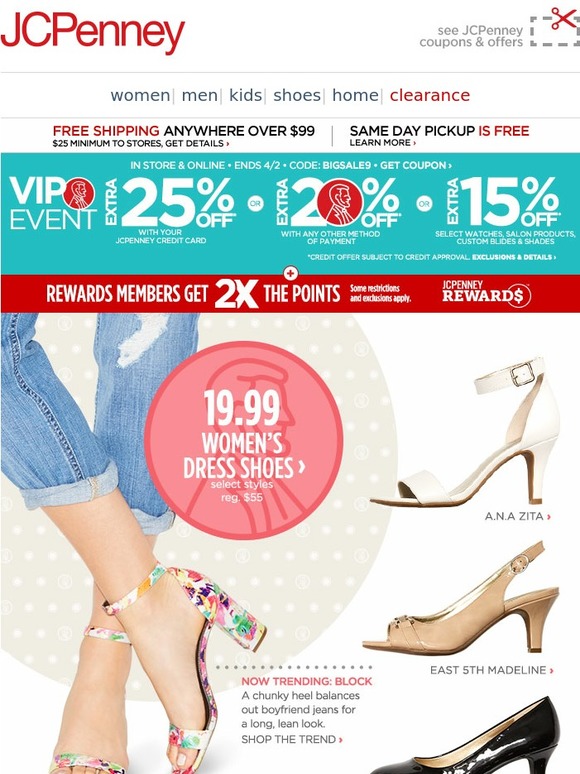Screenshot of the JCPenney Website:

Top Navigation:
- **Logo:** The JCPenney logo in bold red is prominently positioned in the top-left corner.
- **Coupons and Offers:** To the right of the logo, the text "See JCPenney Coupons and Offers" is accompanied by a small scissors icon symbolizing coupons.
- **Navigation Menu:** Beneath, the clickable subheadings include categories: Women, Men, Kids, Shoes, Home, and Clearance.

Promotional Banners:
1. **Shipping and Pickup:** 
   - Text: "Free Shipping Anywhere Over $99. $25 Minimum to Stores. Get details."
   - On the right, "Same Day Pickup is Free" with "Free" highlighted in red, and an arrow with the text "Learn More."

2. **VIP Event Promo:**
   - Text: "VIP Event in-store, online, and for/with code BIGSALE9. Get Coupon."
   - Discounts: "Extra 25% Off with JCPenney Credit Card; Extra 20% Off with Any Method of Payment; Extra 15% Off Select Watches, Selling Products, etc."
   - Additional Banner: A red strip at the bottom reads, "Rewards Members Get Two Times the Points. Some restrictions and exclusions may apply. JCPenney Rewards."

Main Image:
- **Featured Product:** Central to the screenshot is an image of a woman modeling colorful heels.
   - **Description:** She is also wearing ripped, cuffed jeans.
   - **Promotion:** The text "$19.99 Women's Dress Shoes Select Styles Regular $55" is displayed in a red badge.
   - **Highlighted Shoes:** A mini gallery on the right showcases different shoe options:
       1. A white heel labeled **“Ana Sezita.”**
       2. A brown heel labeled **“East 5th Madeline.”**
       3. An unnamed black heel.

This detailed layout captures the JCPenney website's primary elements, highlighting promotional offers, navigation ease, and featured product details.